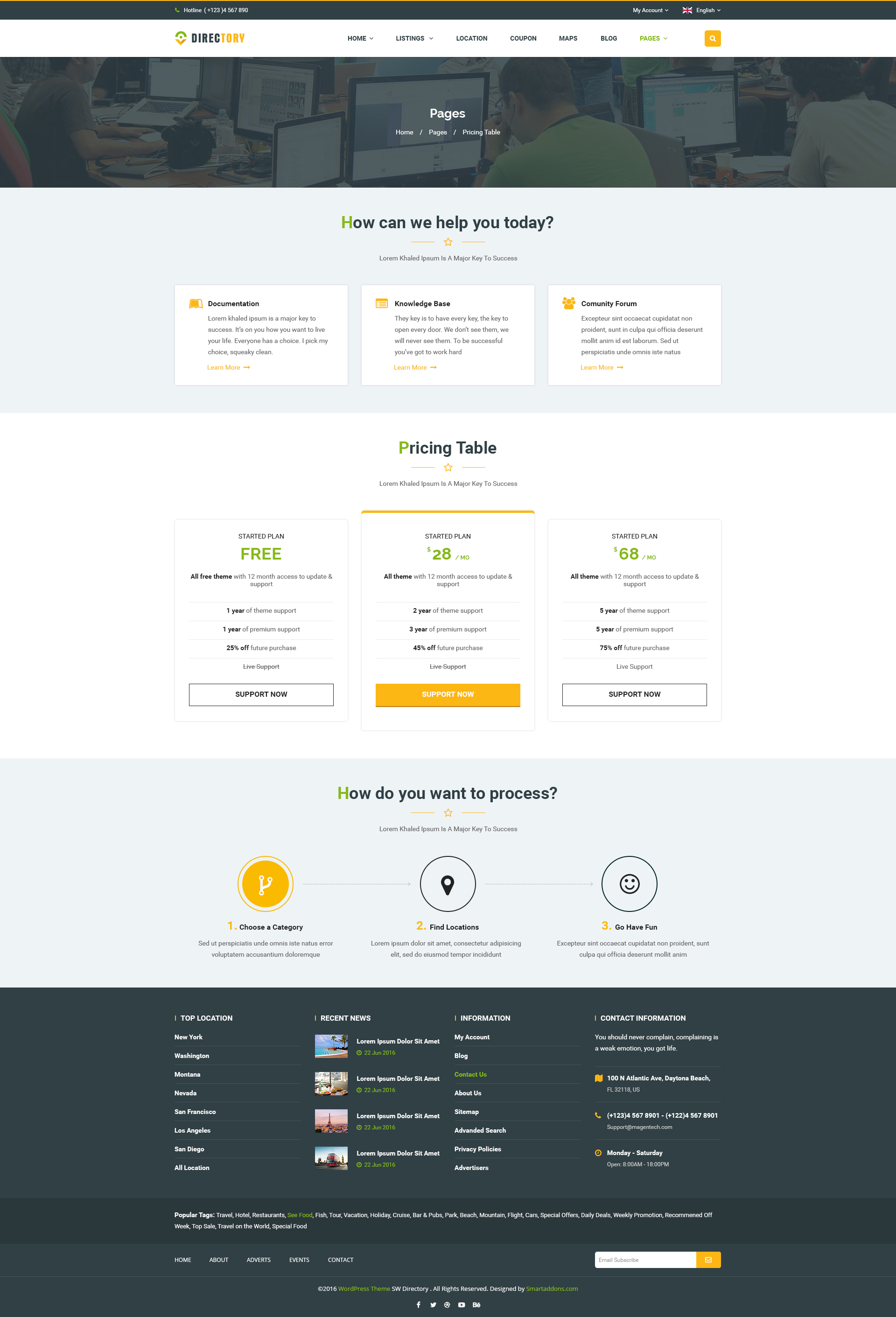The image captures a detailed view of a website interface. At the very top, there is a black banner featuring a small green phone icon followed by the word "Hotline" in white text and a phone number (+123 456 7890).

Below this banner, the site appears to have a navigation menu with capitalized menu items. The word "DIRECTORY" is divided visually, with "DIRC" in black and "TORY" in yellow. The menu items listed are "HOME," "LISTINGS," "LOCATION," "COUPON," "MAPS," "BLOG," and "PAGES." Above this menu, there are options for "My Account" and a language selector showing "English" next to a flag icon.

The main content section features a graphic depicting multiple computer screens and laptops viewed from behind, with a few people visible but only their backs are shown. Below this graphic is a text prompt on either a white or off-white background that reads, "How can we help you today?" This prompt is accompanied by several white squares with labels such as "Documentation," "Knowledge Base," and "Community Forum."

Further down, a larger central square showcases a "Pricing Table." This table lists various plans: a "Free Starter Plan," a "Starter Plan" for $28 per month, and another "Starter Plan" for $68 per month.

Overall, the image showcases a user-friendly and organized website with essential navigation and support elements highlighted for the users.